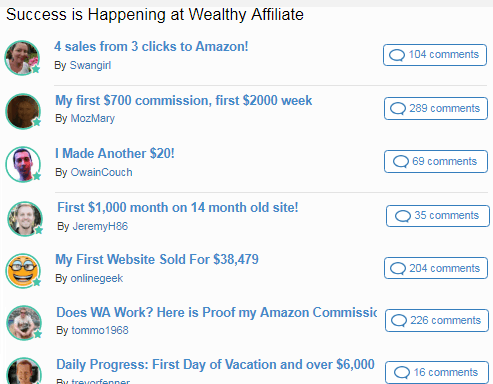### Wealthy Affiliate Success Stories: Community Achievements Showcased

This website screenshot depicts a vibrant community forum, likely from Wealthy Affiliate, focused on sharing success stories and achievements. The interface is clean with a white background. Unlike a mobile or tablet screen, it lacks any top indicators. 

On the left, there's a prominent column structured like an interactive bulletin board, hosting a series of user comments and success stories. Each comment is headed by a title in pale blue text. Beneath each title, the user's name and avatar are displayed to the left, while a clickable blue box to the right shows the number of replies, indicating the presence of active discussions.

The headings of these comments highlight various financial milestones achieved by the users, such as "For Sales from Three Clicks to Amazon," "My First $700 Commission," "First $2,000 Week," and "First $1,000 a Month on a 14-Month-Old Site." More impressive achievements include "My First Website Sold for $38,479" and "Here is Proof of My Amazon Commission," showcasing substantial earnings and successful ventures.

A dark blue or black heading stretches across the top of the page, reading "Success is Happening at Wealthy Affiliate," emphasizing the supportive and triumphant nature of the community. This forum appears to serve as a motivational and informational hub where users can share their journeys and encourage one another in the realm of online business and affiliate marketing.